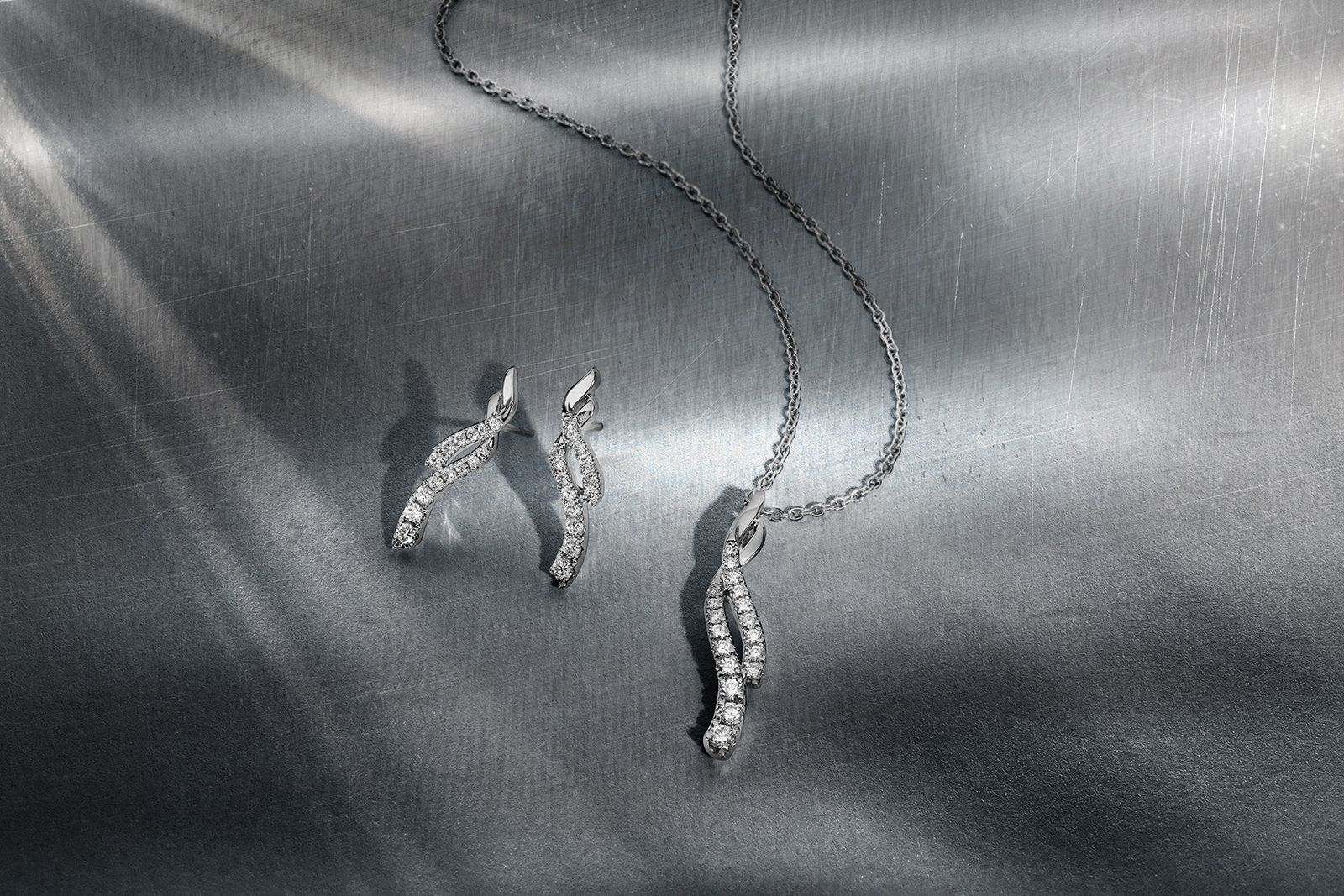In the photo, a sophisticated jewelry set is displayed against a light gray background, with light rays adding a subtle glow to the scene. The set includes a pair of elegant, drop-style diamond earrings and a matching necklace. The earrings feature two curved, asymmetric lines studded with channel-set diamonds—one line is slightly longer than the other, with each boasting around seven to eight diamonds. Complementing these earrings is a necklace that mimics the shape of a free-flowing ribbon or scarf, giving it a graceful, flowing appearance. The pendant, adorned with numerous diamonds, is suspended from a silver chain that lies naturally and fluidly across the surface, echoing the earrings' polished design. The background, which appears to be a lightly textured, possibly scratched stainless steel, adds an industrial yet sophisticated touch to this meticulously arranged jewelry layout.